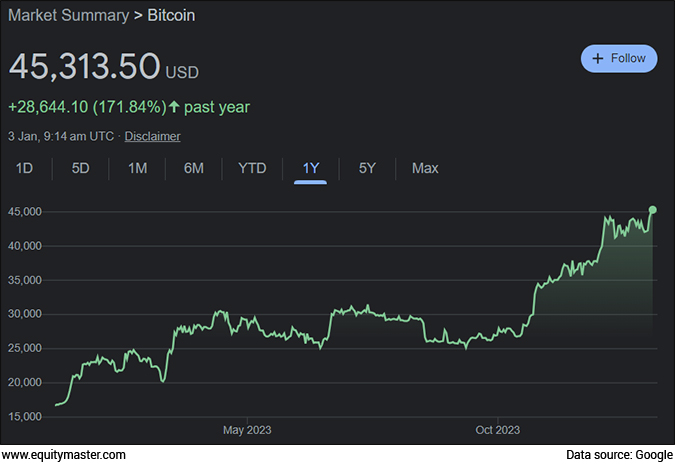The image is a screen capture from the financial website www.equitymaster.com, featuring a predominantly black background. In the lower left corner, the website address is clearly visible. The lower right corner credits Google as the data source with the annotation "datasource: google." Dominating the upper left portion, bold text reads "Market Summary" accompanied by a directional arrow pointing towards information about Bitcoin. Below this header, the current value of Bitcoin is prominently displayed as "$45,350 USD." Additionally, the past year's stock performance is highlighted in green, illustrating positive growth. The main section of the image showcases a detailed chart, which features a green trend line ascending, indicating an upward trajectory in Bitcoin's price trend over the period depicted.